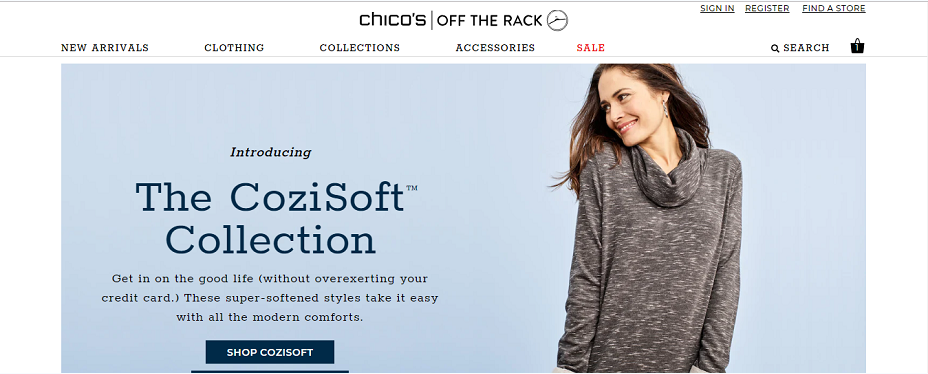The screenshot in landscape mode showcases the homepage of a fashion retailer’s website. 

At the top section, a white horizontal stripe spans across from the upper left to upper right. Located in the upper center is the brand name "Chico's," followed by the tagline "off the rack." In the upper right-hand corner, there are three clickable links: "Sign In," "Register," and "Find a Store," all of which are underlined. 

Below this, a navigation row features headers labeled "New Arrivals," "Clothing," "Collections," "Accessories," and highlighted in red, "Sale." To the far right, a search bar is present beside an icon indicating one item in the shopping cart.

Dominating the center is a large light blue background. On the right side, a light-skinned model with long brown hair—gently blown by a fan—is gazing thoughtfully at the text on the left. She wears a cowl neck, long sleeve brown sweater, accentuated with light makeup and an earring in her left ear.

On the left side, the text reads "Introducing the Cozy Soft Collection," presented above a brief description: "Indulge in the good life without over exerting your credit card. These super soft styles take it easy with all the modern comforts."

Below the description, a prominent blue button invites users to "Shop Cozy Soft," with another partially visible button below it, indicating the page is only partially scrolled down.